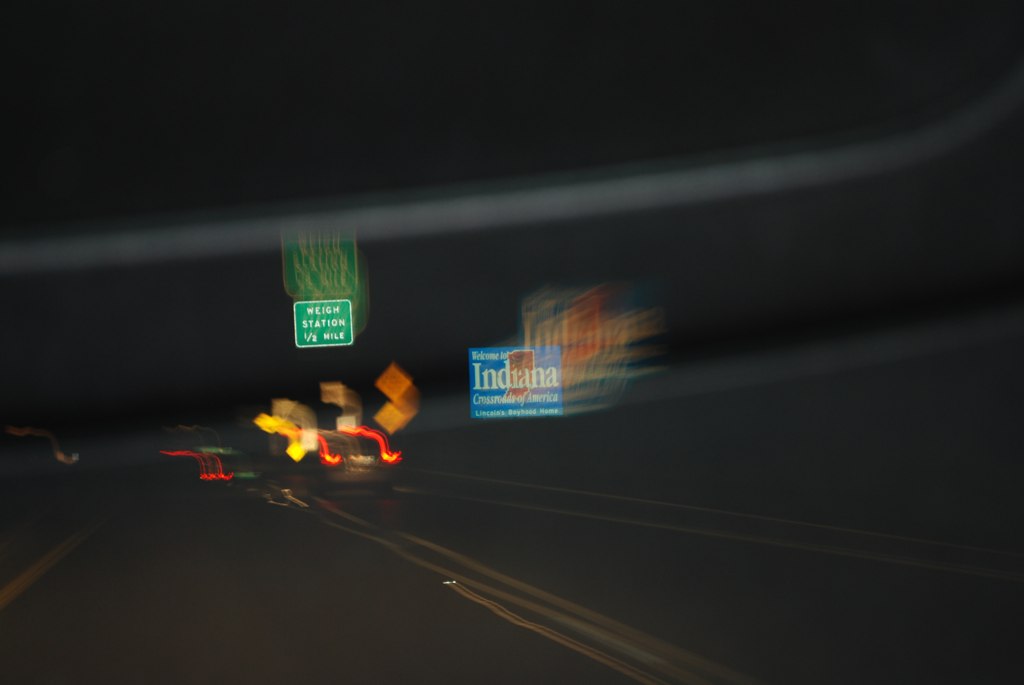The photograph captures a nighttime scene on a highway, likely shot through a vehicle's windshield, adding a layer of reflection. The road appears distorted with a blurry effect. Prominent in the image is a green highway sign on the left that reads "Waystation 1 1⁄2 mile," with an illegible, distorted white text above it. Directly below this, a blue sign warmly welcomes travelers with "Welcome to Indiana" in white letters, accompanied by orange outlines of the state's shape. More white text is present beneath this, but it is unreadable. A ghostly, distorted version of this blue Indiana sign hovers above it, adding to the surreal atmosphere. Double yellow lines trail from the bottom edge to the left side of the image, alongside several road signs – including brown squares and yellow diamonds – scattering across the road. Reflections or possibly papers seem to flutter in the wind, contributing to the image's mysterious and eerie ambiance.